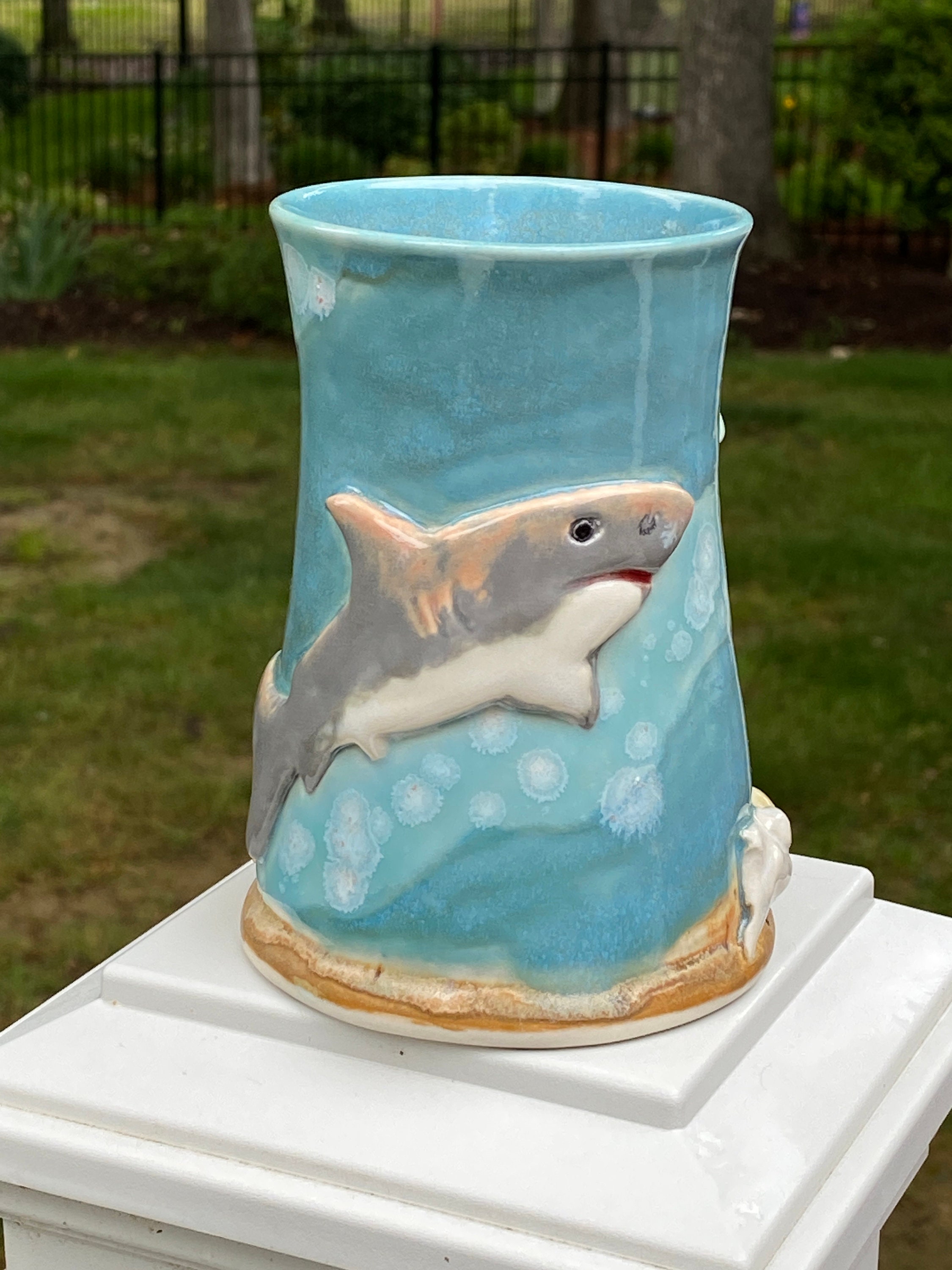This photo captures a custom-made ceramic mug or vase, prominently displayed outdoors. The object, possibly designed as a drinking vessel or flower vase, features a tapered body with a slightly flared top and stands approximately eight inches tall and four inches wide. Its light blue glaze evokes the ocean, complete with a meticulously carved and painted shark in the hues of a great white—including gray, white, and hints of brown. Accentuating the aquatic theme, subtle splotches beneath the shark suggest bubbles in the sea. The vase rests atop a square, white pillar, against the backdrop of a black steel fence adorned with green shrubs and a tree. The lawn in front, marked by sporadic dead patches, completes the serene outdoor setting.